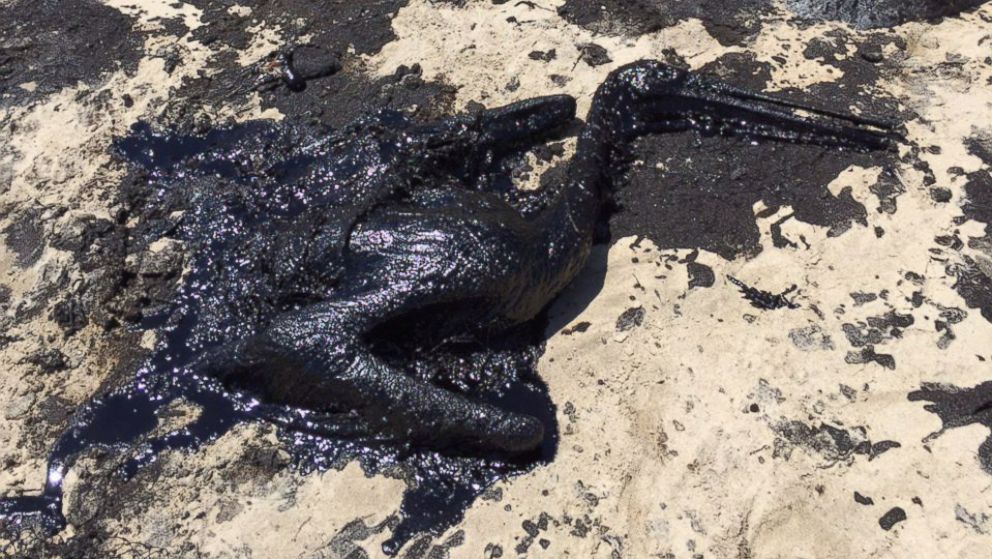The image depicts a grotesque and tragic scene of a large seabird, likely a pelican, entirely covered in thick, shiny crude oil. The bird, unmistakably dead, lies contorted on a sandy beach, with its head resting on its side. The once graceful outline of its long beak and wings is barely distinguishable beneath the black, oily sludge that encases its body. Surrounding the bird, the sand is heavily stained with oil, with large black spots and streams of oil running down to the left corner of the image. Clearly impacted by an oil spill, this heart-wrenching scene highlights the devastating effects of pollution on wildlife and the environment.